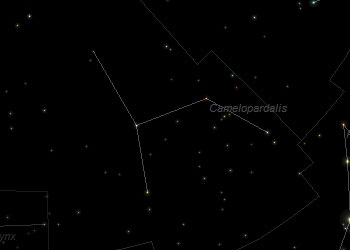This image features the constellation Camelopardalis, set against a solid black background dotted with tiny white speckled stars. The image has a horizontal rectangular shape, slightly wider than it is long, and lacks any bordering. At the center, four connected lines form a trapezoid which is missing the bottom line. One line extends from the upper left corner of the trapezoid down to a small white dot, potentially signifying a star, then continues at various angles to the right. An additional line extends from the top left corner of the trapezoid towards the upper left, creating the impression of a constellation.

Five prominent stars define the constellation, which is described as resembling a camel facing the left side of the image. The name "Camelopardalis" is printed near the upper left line of the trapezoid and also near the center right of the image, indicating its significance. The entire image is rendered in black and white, with the star connections slightly tilted towards the left, likely due to their position in the night sky. There are glimpses of other constellations at the edges—the right and lower left sides of the image—but they are cut off by the image's boundaries, suggesting a broader celestial context just out of view.